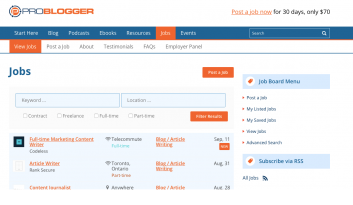The image showcases a small snapshot of the ProBlogger website. The central focus is a job listing section, presumably aimed at bloggers looking for employment opportunities. The interface exhibits a blue and orange color scheme against a white background. Prominently, there's an announcement indicating that job listings are available for 30 days at a cost of only $70. This suggests the platform provides a job board service, facilitating connections between employers and professional bloggers. Due to the small size of the image, finer details remain indiscernible, but the overall impression is of a professional and functional job board.